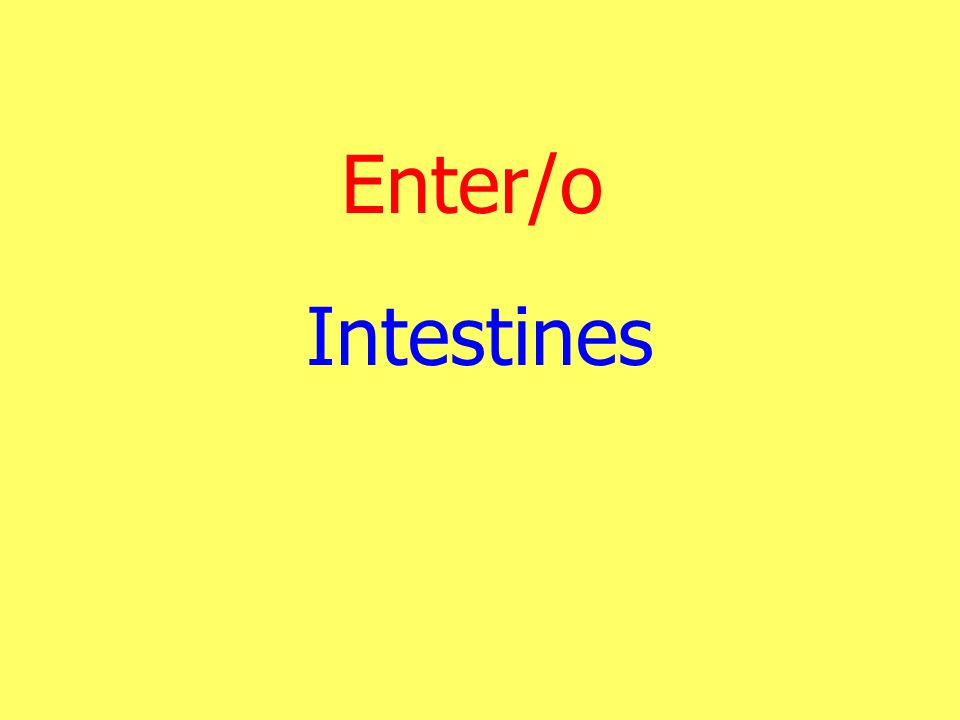The image is a digitally designed graphic featuring a plain, bright yellow background—resembling the color of a Crayola yellow crayon. In the center of the image are two lines of capitalized text. The first line, written in red block letters, displays "ENTER / O." Directly beneath it, in equally sized blue block letters, sits the word "INTESTINES." The graphic is simple with no other elements or text present. The design occupies a rectangle slightly wider than it is tall, with the text centered both horizontally and vertically, suggesting a clean and deliberate layout. The exact purpose of this graphic is unclear, but its minimalistic style and specific choice of text may suggest its use in a scientific or technical context.